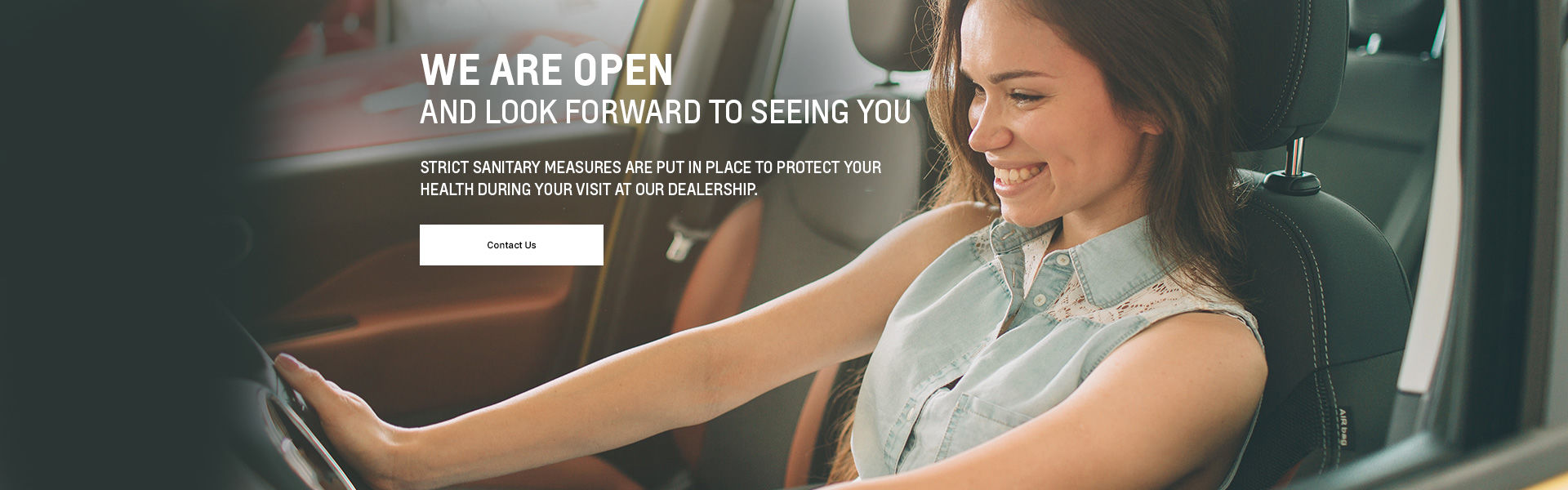This is a vibrant and inviting banner screenshot featuring an enthusiastic female driver. The young woman, who appears to be in her 20s, is captured in a moment of pure joy and excitement, as evidenced by her wide smile. She is dressed in a sleeveless shirt and comfortably seated in a car with sleek black leather seats. Prominently displayed to the left of her is a bold white text that reads, "We Are Open and Look Forward to Seeing You," signaling the dealership's readiness to welcome visitors. Below this welcoming message, in smaller white text, the banner assures customers of their safety with the statement, "Strict sanitary measures are put in place to protect your health during your visit at our dealership." At the bottom of this text block is a white "Contact Us" button, encouraging further engagement.

The background of the webpage continues to showcase the joyful driver, highlighting her arms stretch out and hands gripping the steering wheel, reinforcing the theme of happiness and freedom associated with driving. The overall layout is designed to exude positivity and encourage customers to feel secure and excited about visiting the dealership.